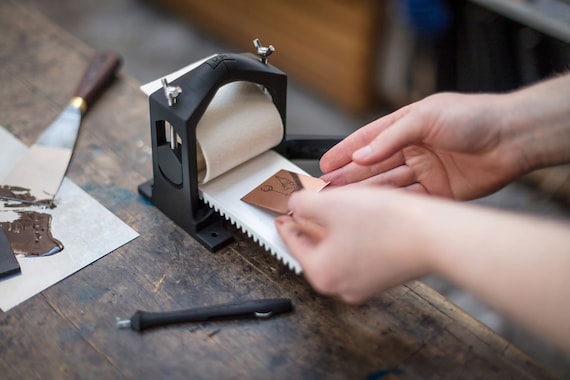In a detailed close-up color photo taken inside a workshop, a black device is clamped onto a round wooden table. The device features two small silver screws at the top and a central slot holding a roll of paper. A pair of hands, coming from the right side of the frame, is meticulously placing a small rectangular object with a picture of a clown holding a balloon onto the paper surface of the device. Adjacent to this setup, in the top left corner of the image, rests a putty knife on a piece of paper, surrounded by a pool of brown putty. The workspace also includes what looks like a small gold or copper plate being positioned onto the white runway of the compact black machine, suggesting that the person is engaged in a craft, possibly printmaking or embossing, where the brown putty or oil might play a role in transferring or enhancing the design. The entire scene conveys a meticulous craft process involving both manual placement and mechanical assistance.